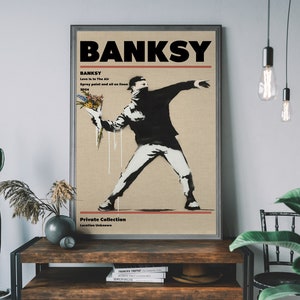This is a detailed photograph capturing a cozy indoor living space, likely a living room, centered around a large poster leaning against a white wall. The poster, with a dark gray border, features a vertical rectangular format with a beige background. At the top, bold black text spells out "BANKSY." Just beneath is a narrow line of red text that's too small to read, followed by three lines of black text, also too small to discern, justified to the left. Dominating the center of the poster is a black-and-white cartoon-style image of a man dressed in a baseball uniform. The man, wearing a black baseball cap, a black long-sleeve shirt, white baseball pants, and black athletic shoes, is depicted in a pitching stance, about to throw a bouquet of pink flowers wrapped in white paper. His left arm is extended outward, his head turned to the right in profile, and his right arm is cocked back in a pitching position. Below this image are a horizontal red line and two more lines of small black text, justified to the left. 

The poster rests on a wooden coffee table, positioned against the wall. To the left of the table, a leafy green fern-like plant in a round gray vase adds a touch of nature to the space. Hanging above the right side of the photograph are two ceiling lights with black cables and sockets, ending in lit light bulbs. Below these lights is a rung-back chair. The coffee table itself has a shelf underneath, which holds a stack of books. The light gray walls of the room complement the warm tones of the wooden furniture, creating a comfortable and inviting atmosphere.